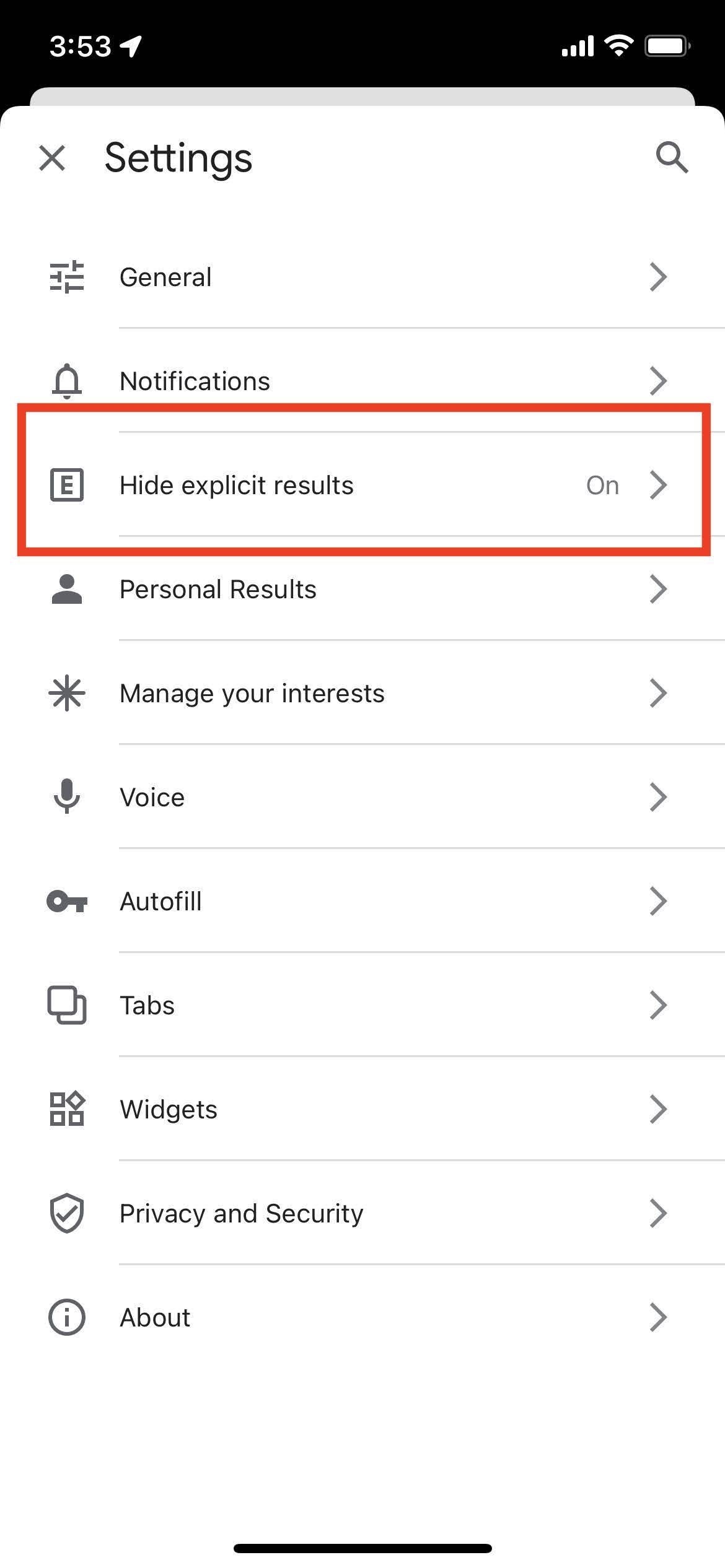The image depicts a cell phone screen showcasing its settings interface. At the top left corner, the time is displayed as 3:53. On the right side of the screen, there are indicators for cellular signal strength, Wi-Fi connectivity, and a fully charged battery. The background transitions from black to white as we move down the image.

At the top left of the white background, there is an 'X' icon, followed by a 'Settings' label to the right. On the far right corner, a search icon is visible. Below this header, the settings options are left-justified, separated by gray lines. The list includes several items, each with a right-facing arrow indicating further submenus. The options listed are: General, Notifications, Hide Explicit Results (currently enabled), Personal Results, Manage Your Interests, Voice, Autofill, Tabs, Widgets, Privacy and Security, and About.

Notably, the "Hide Explicit Results" option is highlighted with a red rectangle drawn using a photo editor, suggesting it may be part of an instructional guide or learning material. This edited annotation indicates the step to access and enable the "Hide Explicit Results" feature. The overall color scheme of the screen includes black, white, gray, and the edited red highlight.

The exact context of these settings is unclear from the image—whether they are for the phone itself or a specific app—since no additional information is provided.